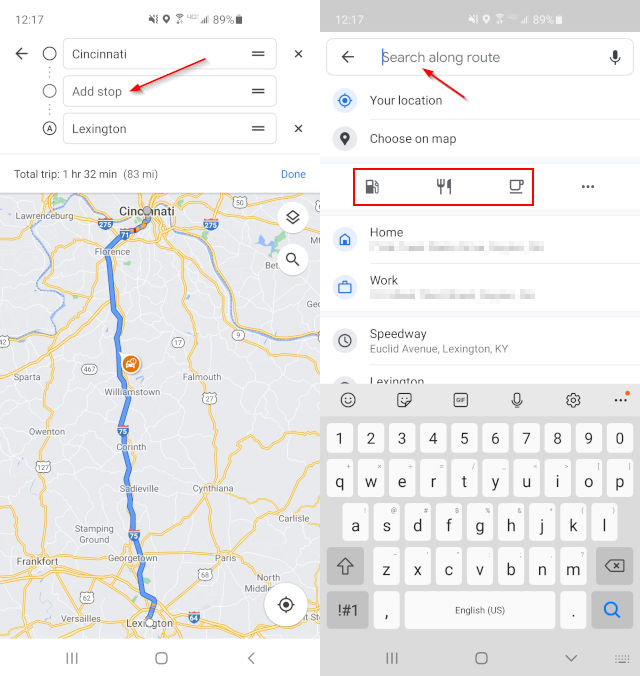The image displays a detailed map interface on a mobile device, showing the city of Cincinnati prominently at the top. The interface is split into two screens side by side, both indicating the time as 12:17 and a battery level of 89%. The top section of the screen includes a title bar labeled "Cincinnati," with an "Add Stop" option and a red arrow pointing towards it. Below this, the map extends to show nearby locations, including Lexington on the right side.

Further down, a search field labeled "Search along route" is highlighted by another red arrow. Below this search field, there are options labeled "Your location," "Choose on map," and icons for gas, food (depicted by a fork and knife), and a cup, all circled in red boxes. 

At the very bottom of the screen, the text "Homework Speedway" appears above a virtual keyboard displaying black letters on mostly white keys, with some keys in gray. The search button, depicted by a blue magnifying glass icon, is prominently visible. The color palette includes yellow, gray, red, blue, green, black, and white, contributing to the map's user-friendly layout and functionality.